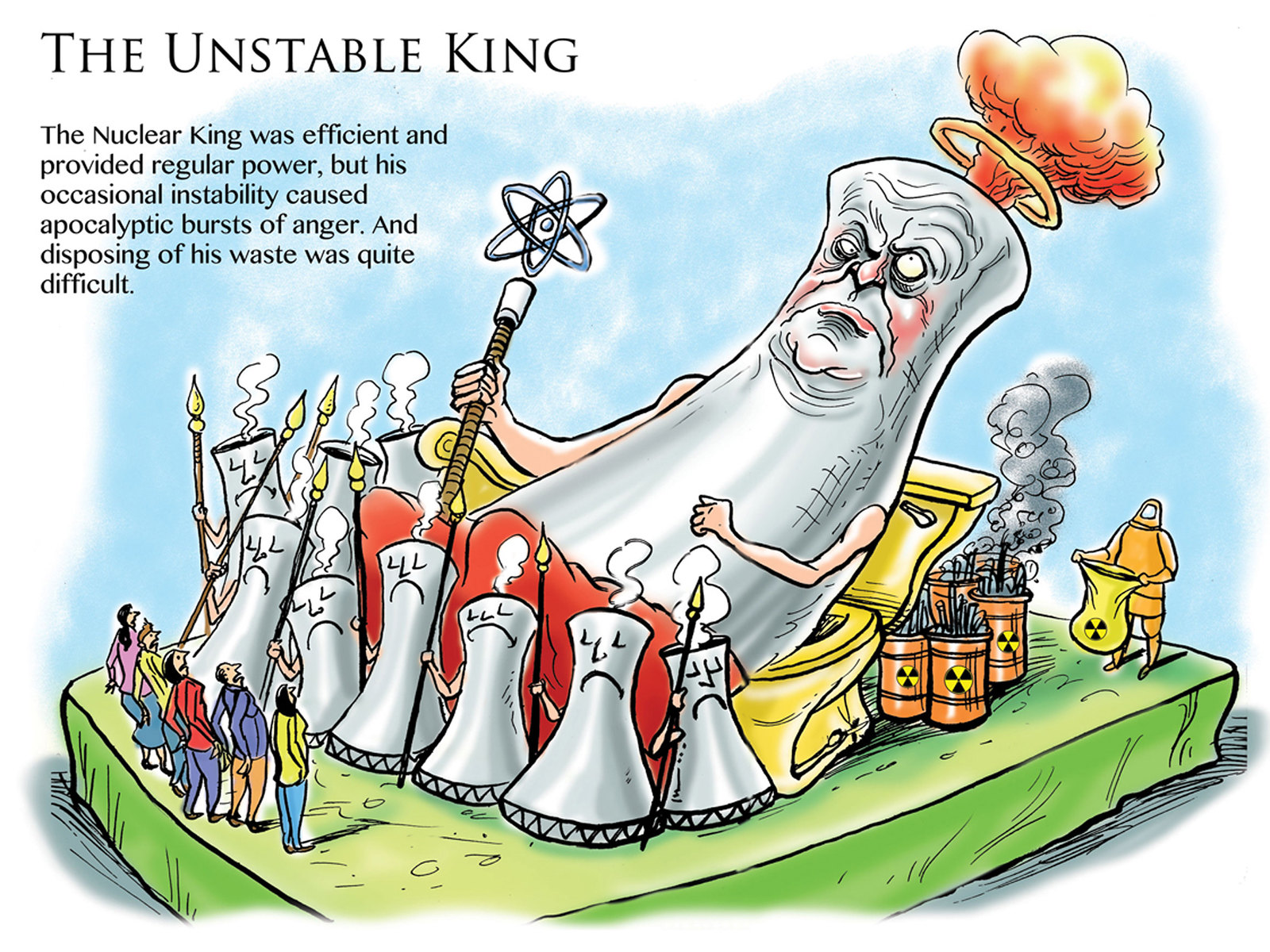The image is a political cartoon illustrating the metaphor of an unstable nuclear king. At the top, the text reads "The Unstable King," and below, it states, "The nuclear king was efficient and provided regular power, but his occasional instability caused apocalyptic bursts of anger and disposing of his waste was quite difficult." Central to the image is a personified nuclear power plant, depicted as an imposing king sitting on a golden throne that cleverly doubles as a toilet, symbolizing the dual nature of nuclear power. Holding a scepter topped with a uranium medallion, the nuclear king has a mushroom cloud billowing from the smokestack atop his head, emphasizing his potential for explosive instability. His face is filled with anger, and he is surrounded by barrels of toxic waste and fumes, with people in radiation suits attempting to clean up the hazardous mess. A parade-like scene unfolds, with nuclear power plant soldiers at his feet and onlookers staring up at the chaotic tableau. The image's color palette includes black, white, orange, yellow, light blue, gray, red, purple, and green, adding vivid contrast to the scene. The artwork lampoons the dangers and challenges associated with nuclear energy, using intricate details to deliver its pointed commentary.